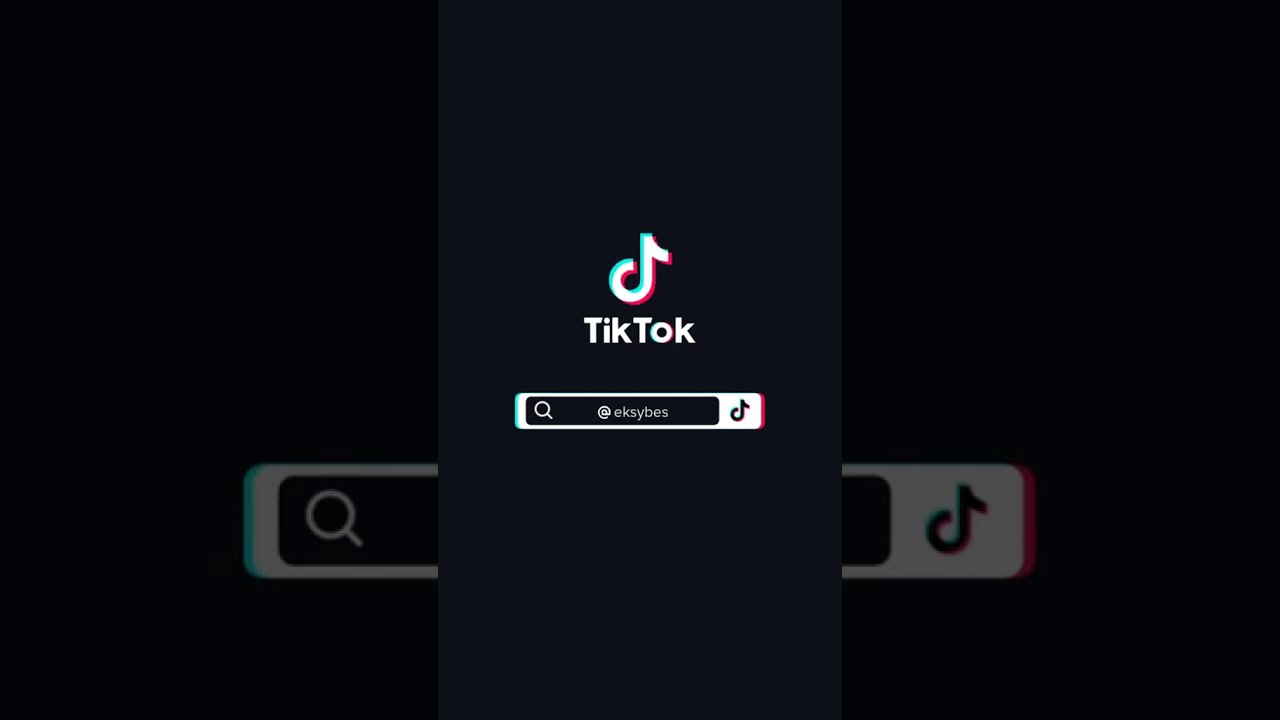The image is a wide rectangular composition featuring a prominent screenshot of TikTok in the center, with darker, close-up images flanking it on both sides. The background is predominantly black, with a hint of deep navy blue. The central screenshot showcases the TikTok logo, a musical note symbol in white with a light blue shadow slightly to the left and a deep pink shadow slightly to the right. Directly beneath this symbol is the word "TikTok" in white text. Below that, there is a white rectangle with curved edges containing a black rectangle with curved edges, displaying the TikTok handle "@EKSYBES." Additionally, at the bottom of the screenshot, there’s a search bar with a magnifying glass icon, indicating that someone is searching for this specific user handle. There are no other pictures, text, or additional context in the image, emphasizing its simplicity and the focus on the TikTok handle.